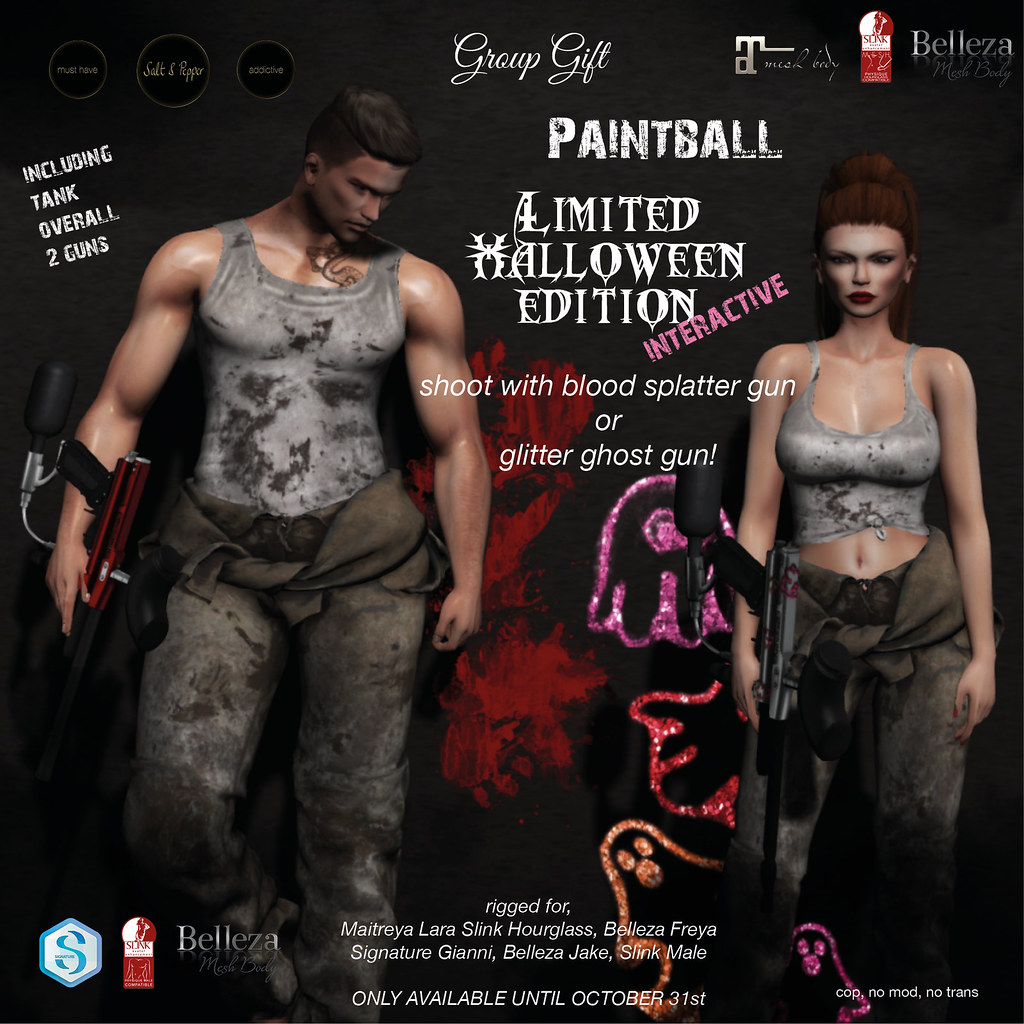The poster is an advertisement for a Paintball event, specifically a limited Halloween edition interactive shoot. It features the option to play with either a Blood Spatter Gun or a Glitter Ghost Gun. The event is available only until October 31st. The poster’s background is dark, and prominently displays a muscular man and a woman, both holding paintball guns. 

The man is tall, wearing a dirty white tank top and dirty pants, with a sweatshirt tied around his waist. He has a tattoo on his chest and upper portion, and holds a shiny, red, and black paintball gun. 

Beside him stands a woman with long red hair, partially tied back into a bun, exposing her large chest and midriff as she wears a tight tank top and dirty gray pants. She too has a paintball gun, and her big red lips are notable.

At the top, the text reads "Group Gift" in white font, followed by "Paintball Limited Halloween Edition: Interactive Shoot with Blood Spatter Gun or Glitter Ghost Gun." Additional details at the bottom of the poster indicate compatibility with various rigs like Maitreya Lara, Slink Hourglass, Belasa Freya, Signature Gianni, Belasa Jake, and Slink Male. It also mentions that it is no-copy, no-mod, and no-transfer. The background includes images of paintball splatters depicting ghosts and blood spatters.